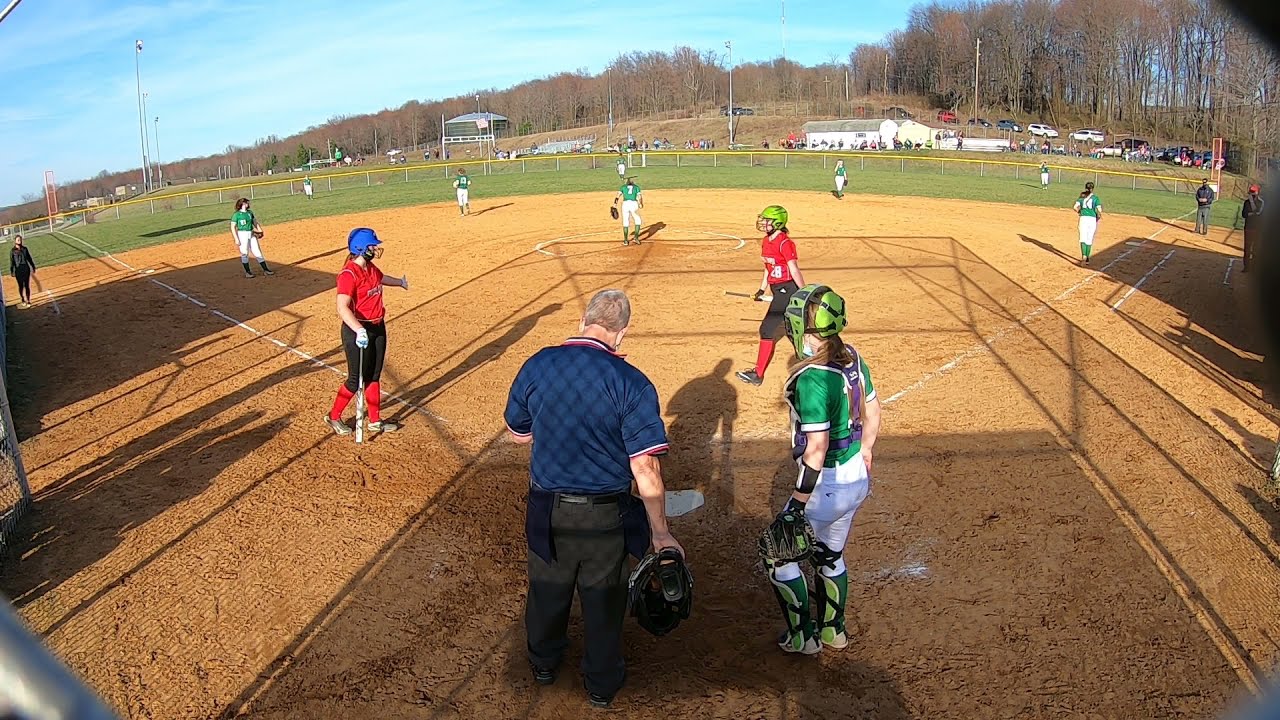Captured from the stands, this horizontally-aligned rectangular image portrays a softball field brimming with anticipation. Central to the framing are the umpire and the catcher, captured slightly from above, suggesting the photographer's vantage point. The umpire, in his short-sleeved blue polo and black pants, holds a helmet in his right hand while presiding over the scene. The catcher, clad in a green top and white pants, has a mitt on their left hand, poised for the next play.

To the left, a batter in a red jersey, green helmet, and black pants walks towards the dugout, exuding a sense of readiness. Nearby, another player, similarly dressed in a red jersey and black pants but donning a blue batter's helmet, prepares to step up to the plate. The outfield team wears green uniforms paired with white pants, set against a backdrop of barren or possibly brown-tinged trees, suggesting an early spring day. The striking blue sky adorned with white, feathery clouds crowns the scene with serene beauty.

The field itself transitions from a dirt infield to a grassy outfield, bordered by a home-run fence. Beyond the fence, a tableau of hills and dry terrain extends into the distance, indicative of a dry season before the revitalizing rain. The scene is bathed in sunlight, the shadows hinting at a late afternoon glow. The players appear in a moment of pause, hands on hips and bats in hand, awaiting the next play in this slice of outdoor sports life.